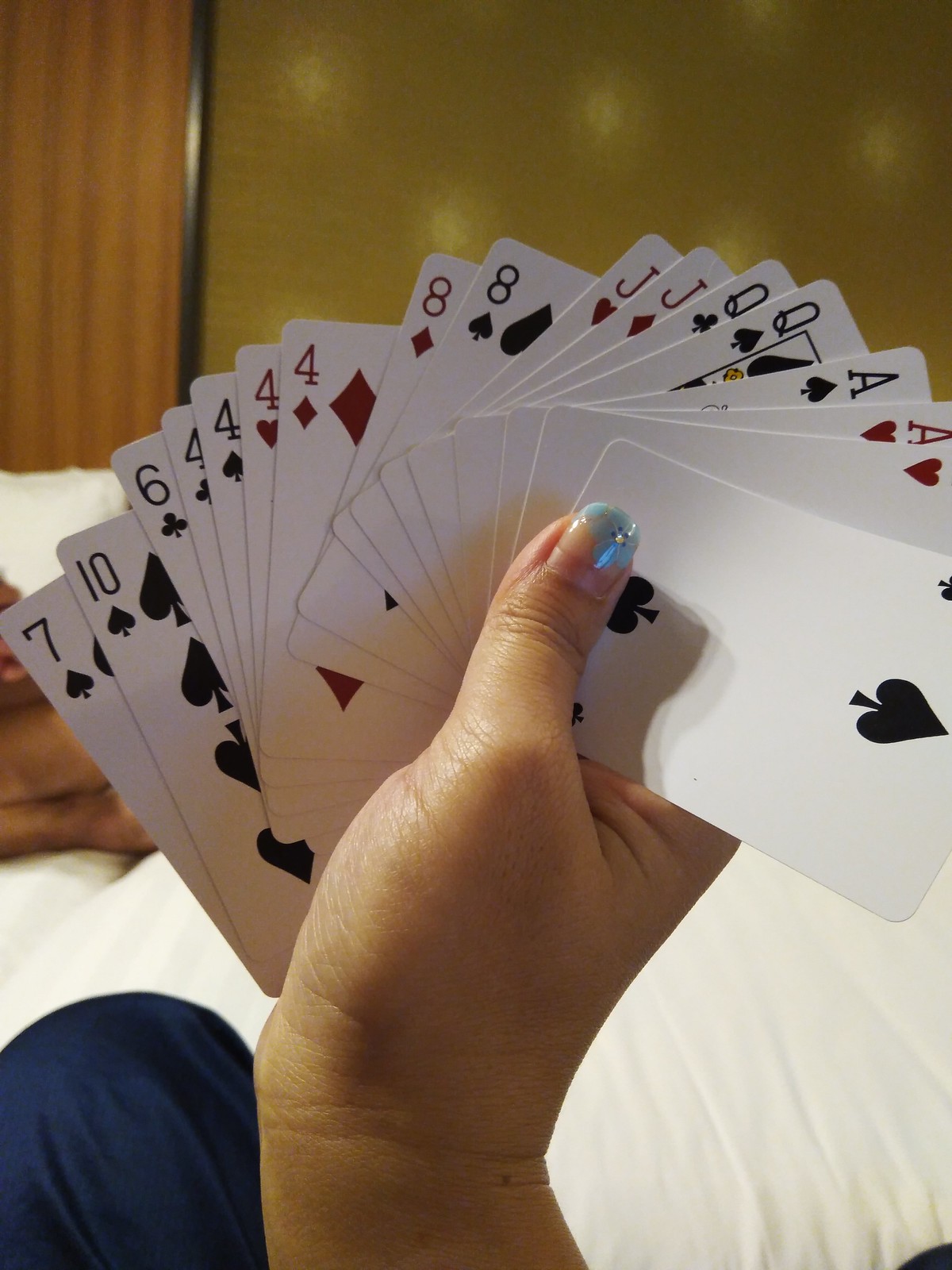A person is seated on a bed with white covers, holding a fanned-out deck of playing cards. Their nails are painted, with a light blue flower design featured prominently on their thumb. The individual appears to be wearing dark blue pajamas, visible in the lower left corner of the image. In the background, there are indistinct hands or feet and the setting includes a green wall alongside a wooden wall.

The playing cards are arranged neatly in their hand and include the following:
1. Seven of Spades (black)
2. Ten of Spades (black)
3. Six of Clubs (black)
4. Four of Clubs (black)
5. Four of Spades (black)
6. Four of Hearts (red)
7. Four of Diamonds (red)
8. Eight of Diamonds (red)
9. Eight of Spades (black)
10. Joker
11. Queen of Spades (black)
12. Ace of Spades (black)
13. Ace of Hearts (red)

Two additional cards, presumably a heart and a spade, are partially visible but obscured.